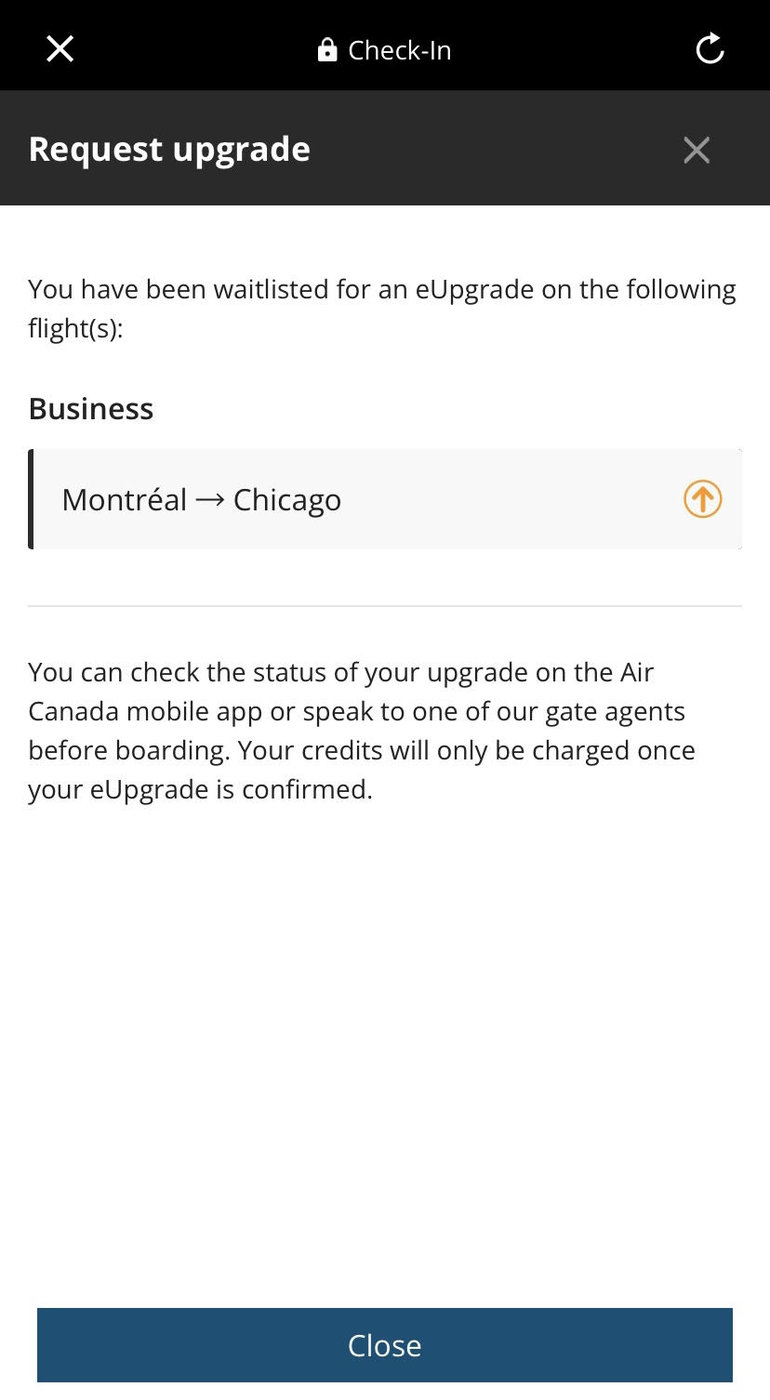The image appears to be a screenshot from a mobile device, possibly a phone or tablet. At the top left corner, there's a black bar featuring a white "X" icon followed by a lock icon. Next to these, the text "Check-In" is displayed, accompanied by a circular refresh arrow icon. To the right of these elements, the phrase "Request Upgrade" is shown in white font, followed by another white "X" icon.

The main content area has a white background with black text that reads: "You have been wait-listed for an eUpgrade on the following flights." Below this text, there is information specifying the upgrade type and flight route. The word "Business" is displayed, followed by "Montreal → Chicago," indicating a flight departing from Montreal and arriving in Chicago. 

An orange circle with an upward arrow inside is placed next to the flight information. Additional text informs the user: "You can check the status of your upgrade on the Air Canada mobile app or speak to one of our gate agents before boarding. Your credits will only be charged once your eUpgrade is confirmed."

At the bottom of the screen, there is a blue button with white text that says "Close."